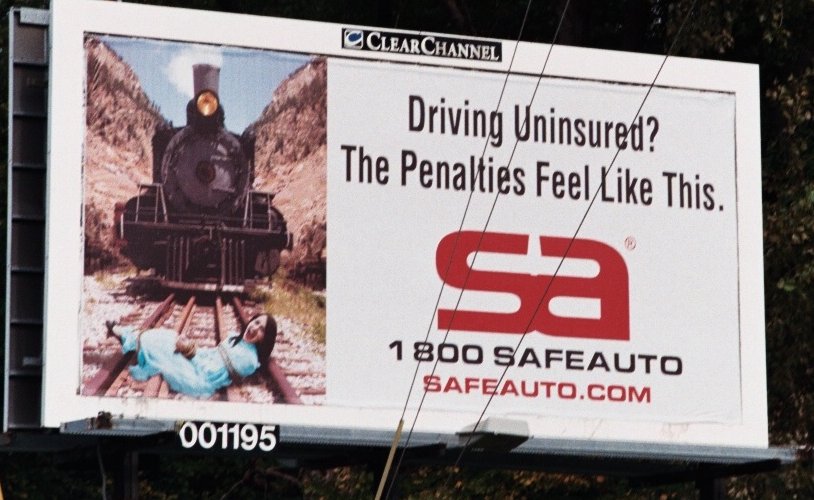This detailed image features a roadside billboard owned by Clear Channel, prominently noted at the top edge of the board. The billboard is encased in a white border and has an upward-facing light fixture at its base for illumination. The advertisement displayed on the billboard is for the car insurance company, Safe Auto. 

On the left side of the advertisement, a dramatic scene is depicted with a train and a woman tied up and lying on the tracks, implying an impending danger. This striking visual is paired with the bold black text: "Driving uninsured? The penalties feel like this." 

The Safe Auto logo, consisting of an "S" and "NA" with a copyright symbol, is positioned nearby. Below the logo, the contact information is displayed in black text: "1-800-SAFE-AUTO." Just underneath this, the company's website, "safeauto.com," is printed in red.